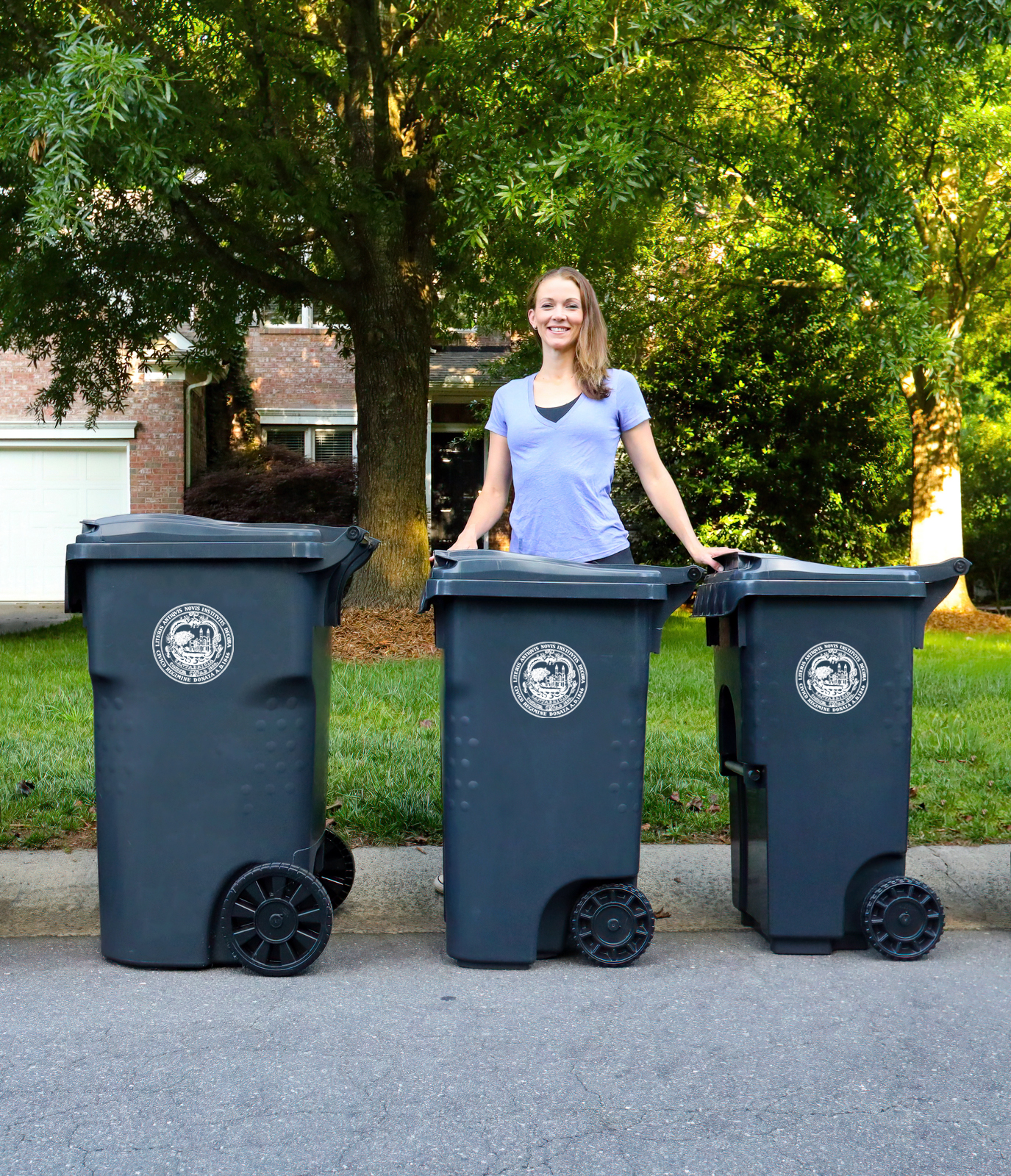In the image, a fair-skinned woman with medium-length light brown hair stands in front of a lawn with green grass. She is positioned behind three black trash bins aligned in a row on a road. Each bin bears a white logo depicting an anteater facing left, encircled by a blue ring, with small, illegible text around it. The woman, smiling at the camera, wears a light blue short-sleeved t-shirt over a dark blue tank top, and her hands rest on the central and right bins. The bins differ slightly in size and wheel design: the left, largest bin has big black wheels; the central bin appears to have dual-layered wheels; and the right bin features ridged wheels. In the background, there are several trees, including a tall one, a portion of a house with dark brown walls and a white garage door, as well as some scattered leaves on the ground.